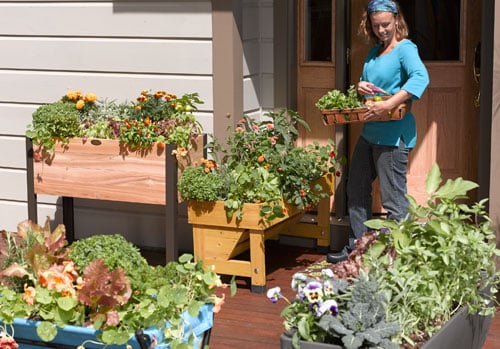The image depicts a woman in a gardening scene set upon a wooden deck, possibly her front porch. She is wearing a blue t-shirt with three-quarter sleeves, a blue headband, gray pants, and black gardening shoes. Her shoulder-length blonde hair is styled in loose waves. The woman is holding a basket filled with various plants, including what seem to be herbs, vegetables like lettuce, shallots, and maybe tomatoes or peppers. 

In the background, a door is slightly ajar, suggesting she has just stepped out of her house. The deck is adorned with a variety of planters and flowerbeds, some elevated on tables. These planters, which include blue and gray containers, are brimming with mostly green leafy vegetation. Among the greenery, there are bursts of color from marigolds with shades of orange and gold, and pansies that are purple and yellow. The overall scene conveys a serene moment of outdoor gardening, with the woman tending to her plants amidst a variety of green leafy vegetables, herbs, and a scattering of colorful flowers.